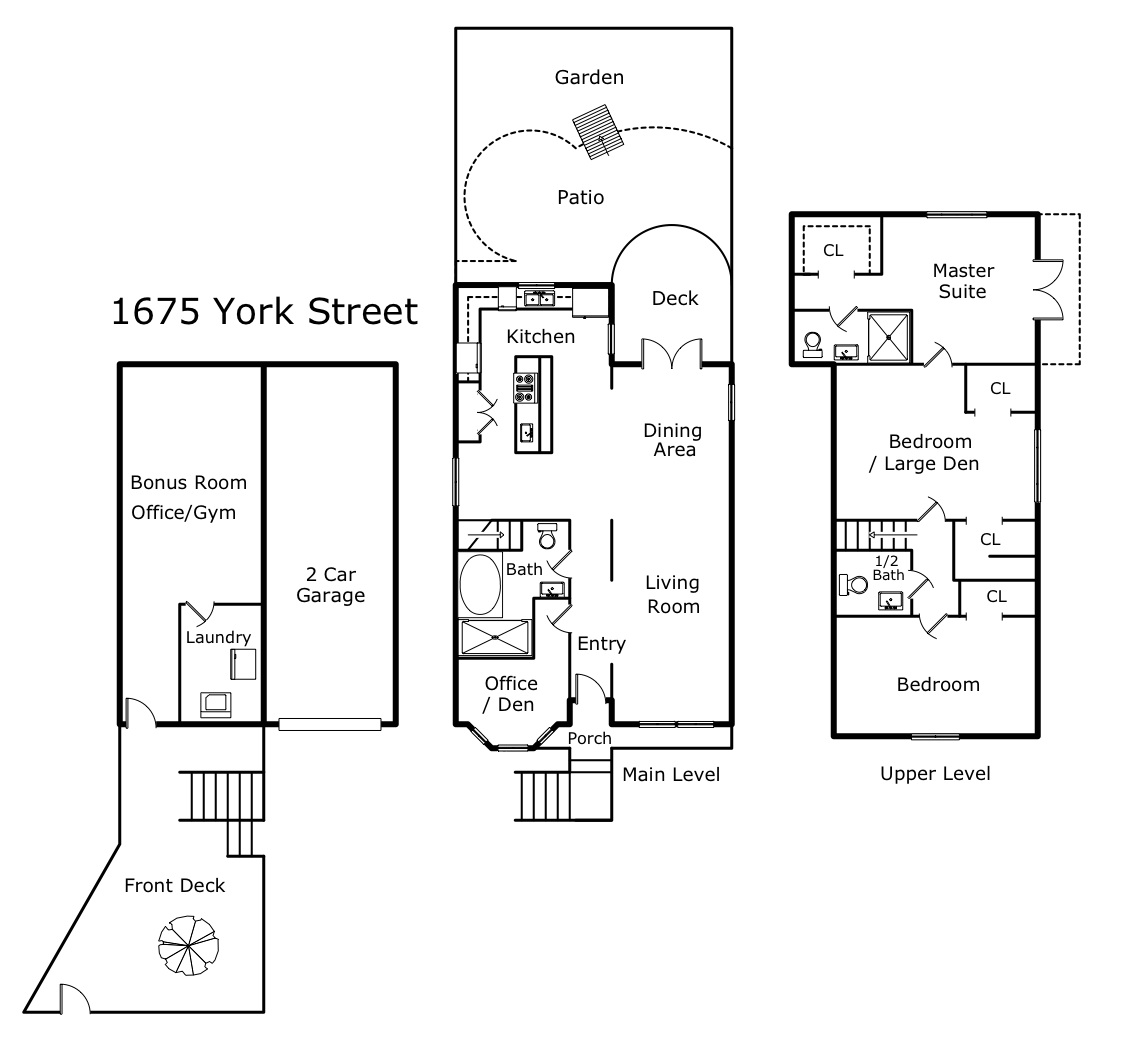Detailed architectural blueprint for 1675 York Street. 

The blueprint, laid out on a white background, spans across the document without being confined by a rectangular border. Key details, such as "1675 York Street," are prominently displayed in bold black letters on the left side. The design is delineated with sections in various shades of boldness, offering clarity on different rooms and levels of the building.

**Exterior and Main Levels:**
- **Front Deck:** Situated at the lower left, providing access to the house.
- **Laundry Room:** Located just above the front deck entrance.
- **Bonus Room/Office/Gym:** Adjacent to the laundry room.
- **Two-Car Garage:** Positioned next to the bonus room, accessible from the exterior.

After the main entrance:
- **Porch and Entryway:** Leading into the main level.
- **Office/Den and Bathroom:** Placed to the right upon entering.
- **Living Room:** Centrally located, directly above the entryway.
- **Dining Room:** Situated to the left of the living room.
- **Kitchen:** Adjacent to the dining room.
- **Deck and Patio/Garden:** Accessible from the dining room, leading to exterior relaxation spaces.

**Upper Level:**
- **Bedrooms and Bathrooms:**
  - Multiple bedrooms are mapped out with associated bathrooms.
  - A closet is highlighted for each bedroom.
- **Large Den:** Situated further up, flanked by additional closets.
- **Master Suite:** Located towards the rear, featuring an expansive layout that includes a bath area and a large closet.

Overall, the blueprint provides a comprehensive view of the structure’s layout, from the functional areas like the garage and laundry room to the more leisurely spaces like the patio and garden. The design ensures a harmonious flow between living, working, and recreational areas.